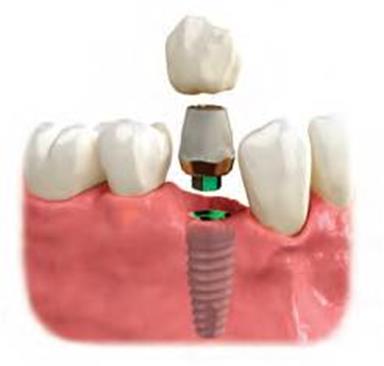The image is a detailed, digitally-created diagram set against a plain white background, illustrating a dental procedure. The focus is on a section of gums and teeth with a clear 3D perspective that suggests the installation of a dental implant. In the center, a screw is being placed into the pink gums, preparing for the attachment of a crown or cover. Surrounding the implant site are four natural teeth—two on either side—highlighting their position in the gum line. The fake tooth appears to be made of porcelain or a similar material. The colors in the image include white, off-white, green, pink, and gray, and the composition suggests it is designed for educational purposes, likely intended for a dental school or medical pamphlet. There is no text in the image, and the detailed rendering emphasizes the procedural steps of dental implantation.